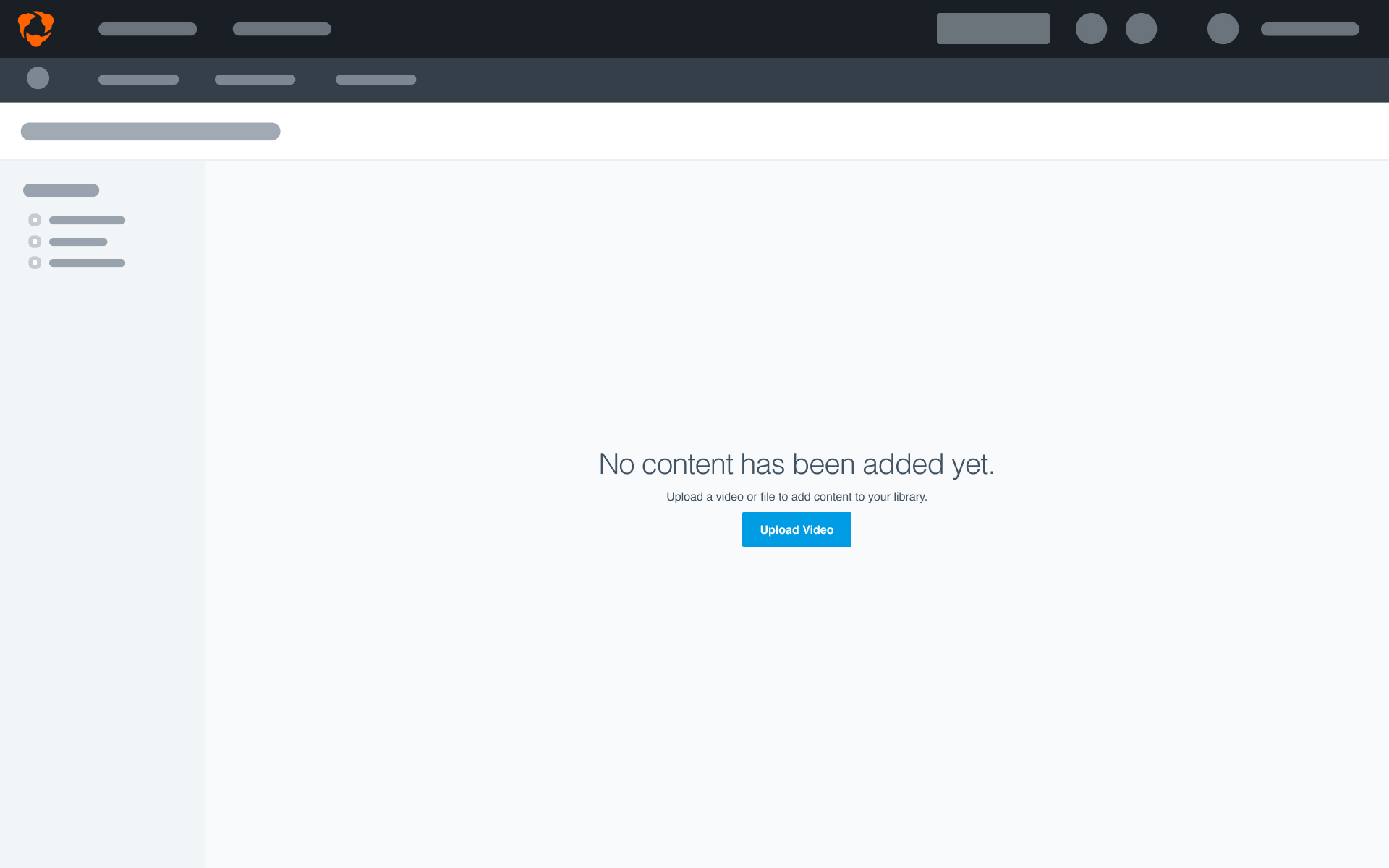The image depicts a minimalistic website template with a structured layout, primarily composed of various grayscale placeholder elements. The top section of the page features a black header bar, adorned with blank gray placeholders, indicating where key navigational or branding elements would typically reside. Directly below this is a lighter black navigation bar, also containing four grayed-out placeholders arranged horizontally, likely intended for important links or features.

Beneath these header sections, the main body of the template is a light gray area. At the top of this section lies a dark gray strip, clearly designed to function as a header for a search bar. On the top left side of the page is a vertical column running down the entire length, filled with additional placeholders meant to serve as categories or navigation links.

The main content area to the right of the vertical column remains largely empty, featuring a prominent message in the center: "No content has been added yet," displayed in large black letters. Below this message, instructions prompt the user to "upload a video or files to add content to your library." Finally, a blue button labeled "Upload Video" suggests the intended user action. Overall, the template is simplistic and awaits further content to bring it to life.